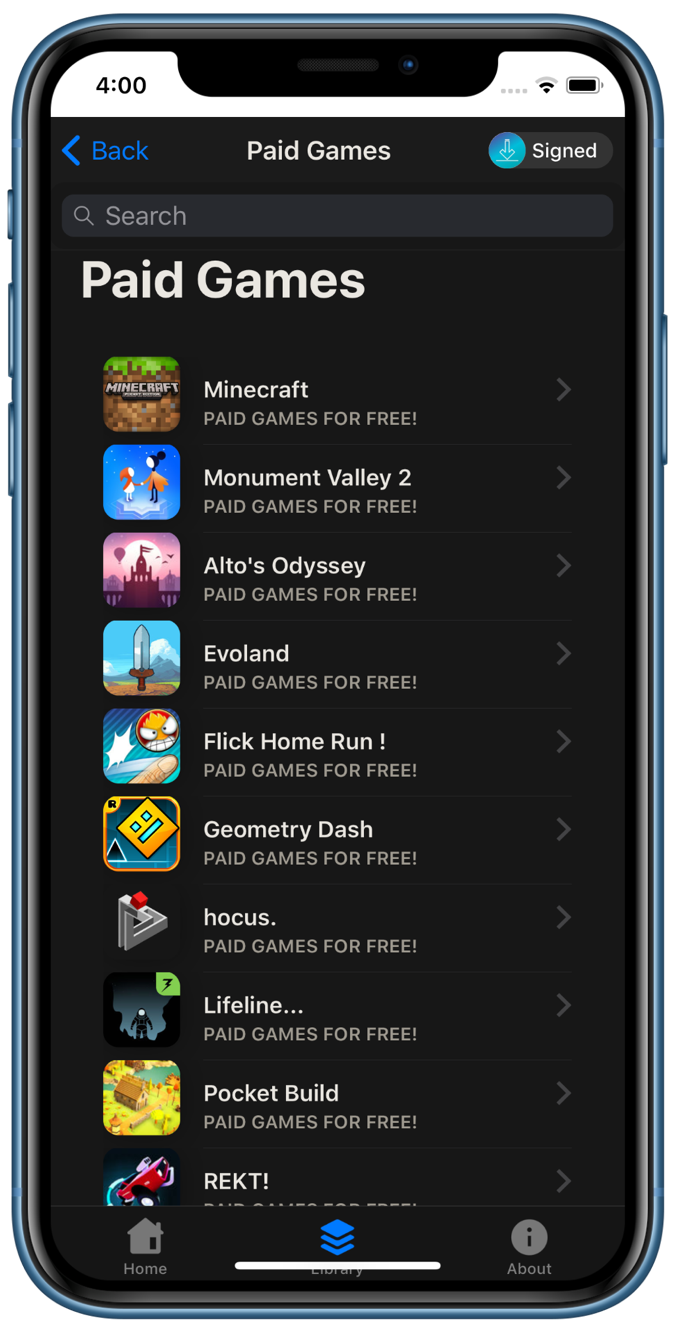The image features an iPhone-style cell phone with a metallic blue exterior and a black border surrounding the screen. At the top of the screen, the front-facing camera is encircled by a white border. The status bar displays the time "4:00" on the left, while the right side shows the battery icon, Wi-Fi signal, and four dots indicating network strength.

The screen's interface shows a black background with a blue arrow pointing left labeled "Back" at the top left. In the center is the title "Paid Games" in white capitalized text. On the right, there is a blue circle with a downward arrow next to the word "Signed" in white capitalized text.

Below this header, there is a search bar. Underneath the search bar, the words "Paid Games" are prominently displayed in bold, capitalized letters. The following is a list of paid games, each name capitalized:

- Minecraft
- Monument Valley 2
- Alto's Odyssey
- Everland
- Flick Home Run
- Geometry Dash
- hocus.
- Lifeline
- Pocket Build
- REKT!